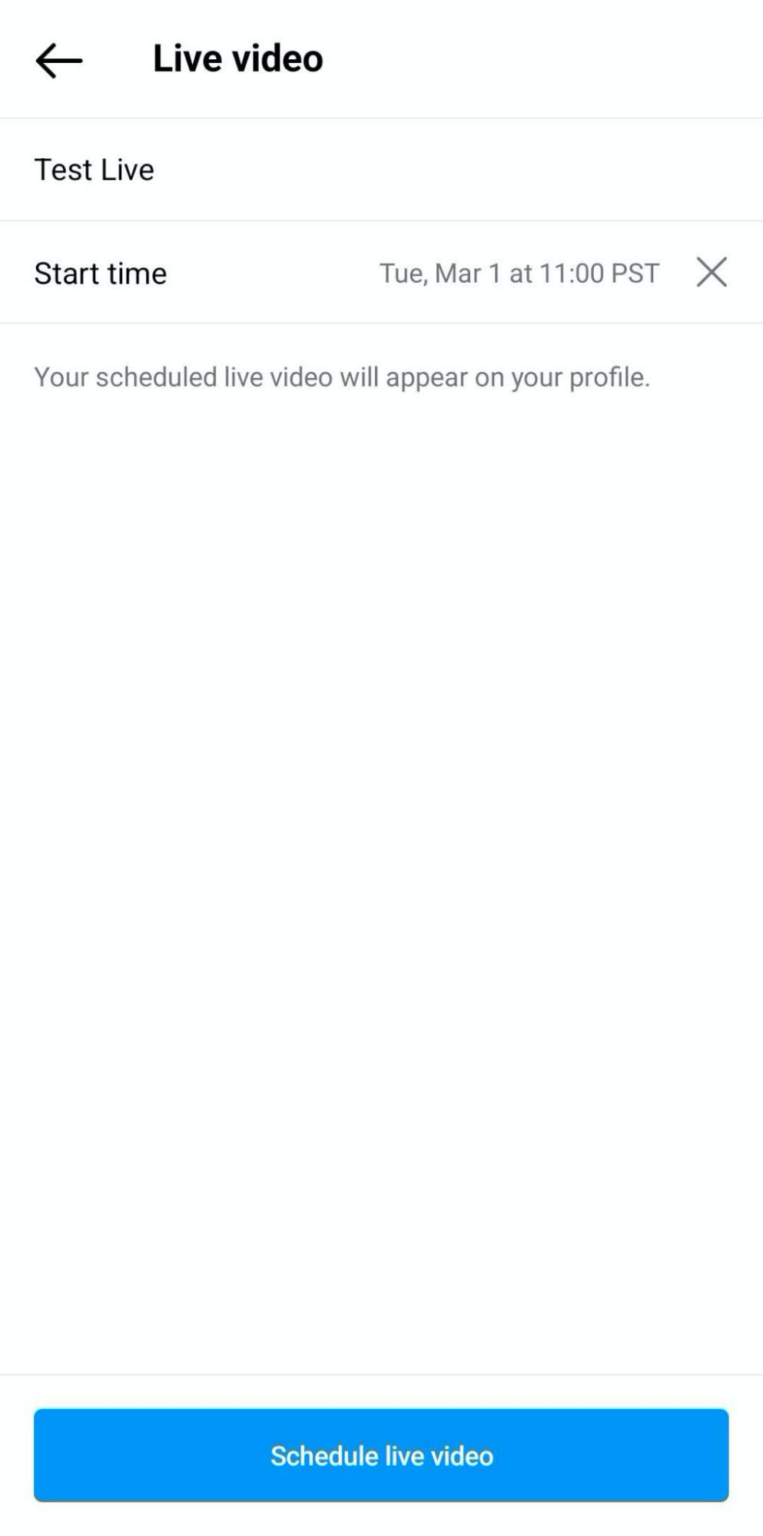This image is a screenshot of a website accessed via a smartphone, evident from its narrow and elongated format. At the top of the screen, there's an arrow icon accompanied by the text "Live Video." Below this header are two listings: "Test Live" and "Start Time." Adjacent to "Start Time" are the details "Tuesday, March 1 at 11 PST" in gray letters, indicating Pacific Standard Time. Next to this timestamp, an 'X' icon suggests the option to delete or modify the scheduled start time. Further down, a message reads, "Your Scheduled Live Video Will Appear on Your Profile," signifying that a live video has been planned for Tuesday, March 1 at 11 a.m. At the very bottom, a blue bar with white text reads "Schedule Live Video," implying that the user needs to click this button to confirm and officially schedule the live video.